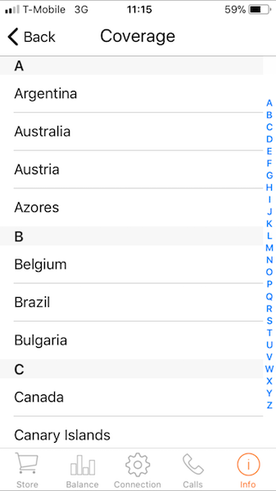This is a detailed screenshot of a cell phone service provider's app, specifically displaying the "Coverage" tab. At the top of the interface, there's a "Back" button on the top-left corner, accompanied by a backward-pointing arrow. Prominently centered at the top, the word "Coverage" is displayed in large black letters, denoting the active section.

Beneath this heading is an organized, alphabetical listing of countries sorted into distinct categories. Each alphabetical category is separated by a wide, rectangular gray divider bar. For example, the letter "A" is listed first in one of these bars, followed by countries such as Argentina, Australia, Austria, and the Azores. 

The letter "B" in another identical gray bar comes next, listing Belgium, Brazil, and Bulgaria beneath it. Following this, the letter "C" is presented in a similar gray bar, with Canada and the Canary Islands listed below.

At the bottom of the screenshot, there are navigation icons arranged in a row: "Store," "Balance," "Connection," "Calls," and "Info." While most icons are in light gray, indicating they are inactive, the "Info" icon stands out in red, highlighting its active status.